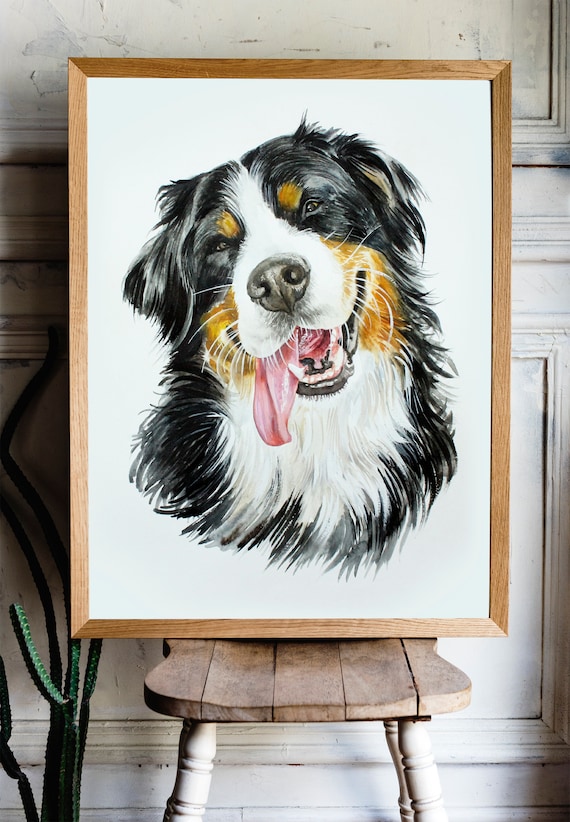A realistic, vertically-oriented color photograph captures a cozy indoor setting with a weathered white wooden wall and paneling as the backdrop. In the left corner, a slender cactus plant, about two to three feet high, adds a touch of greenery to the scene. At the bottom center, the white legs and slightly faded wooden seat of a chair are visible, drawing the eye to the centerpiece: a framed portrait of a dog perched on the chair. The portrait, encased in a light wooden frame, features no text and showcases the dog from the shoulders up against a plain white background. The dog, likely a border collie or St. Bernard mix, has expressive brown eyes and a joyful demeanor, with its head slightly tilted to the left and its tongue playfully hanging out. The dog's fur is a striking combination of black, light brown, and white—black fur predominates, with light brown around the face and shaggy brown "eyebrows," while white fur highlights the nose, chest, and ruff. The overall composition evokes a sense of warmth and happiness.